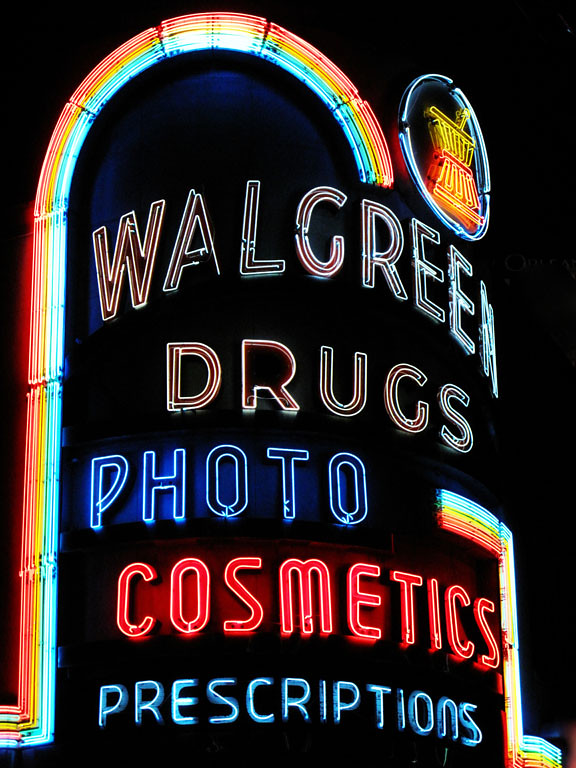This is a nighttime photo of a very old neon sign for Walgreens. The sign prominently displays "Walgreen Drugs" in white neon lighting, followed by "Photo" in blue, "Cosmetics" in red, and "Prescriptions" in blue. The entire sign is well-illuminated against a black background. A distinct feature of the sign is a colorful, rainbow arch consisting of red, yellow, blue, and green lines, which starts from the bottom left and curves up to the top of the sign, resuming from a gap at the top and continuing down to the bottom right. At the top right corner, there is a symbol resembling a medical vessel with a rod and a tip, set against a blue circle.